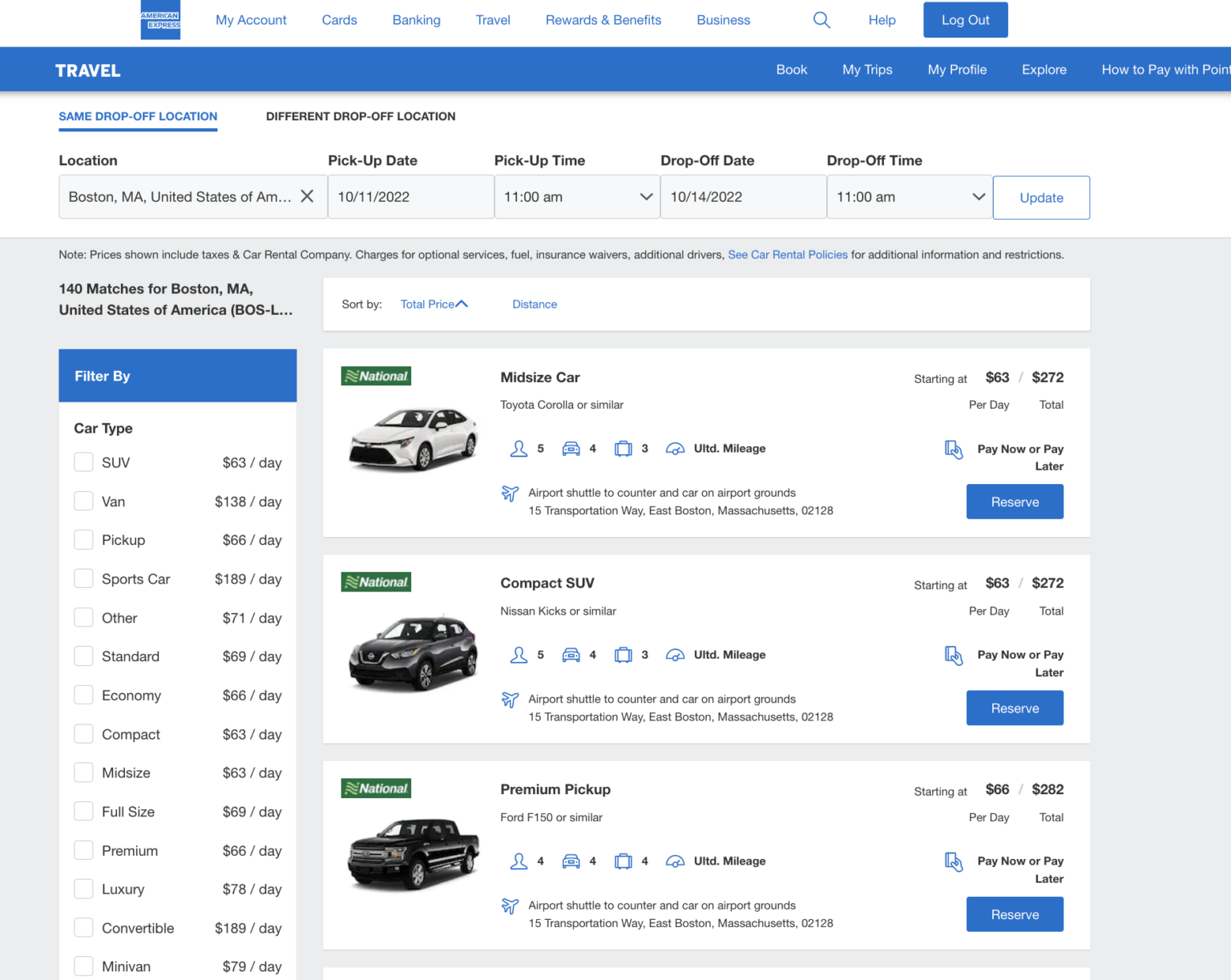The image captures a web page from a car rental selection app, primarily featuring a white background with blue accents. At the top of the page, a blurred blue box with white letters possibly indicates "American Express." Adjacent to this, within a white-bordered section, are blue-highlighted navigation options: "My Account," "Cards," "Banking," "Travel," "Rewards and Benefits," "Business," a search magnifying glass icon, a "Help" button, and a blue "Logout" button with white lettering.

Below this header, there is a rectangular blue box displaying white text, with "Travel" on the left and "Book," "My Trips," "My Profile," "Explore," and "How to Pay with Points" aligned to the right. Further down, two options are presented on a white background: "Same Drop-Off Location" and "Different Drop-Off Location." Users can choose their location, pick-up date and time, drop-off date and time, each accompanied by drop-down carets and an "Update" button in white and blue.

Beneath this section, lies a gray box featuring various options. On the left is a "Filter By" column, listing car types and different vehicle rates. On the right side, various car options are displayed, including "Midsize Car," "Compact SUV," and "Premium Pickup," with all vehicles listed under the "National" company complete with accompanying images. Each vehicle option includes a blue "Reserve" button with white font, enabling users to select their desired car.